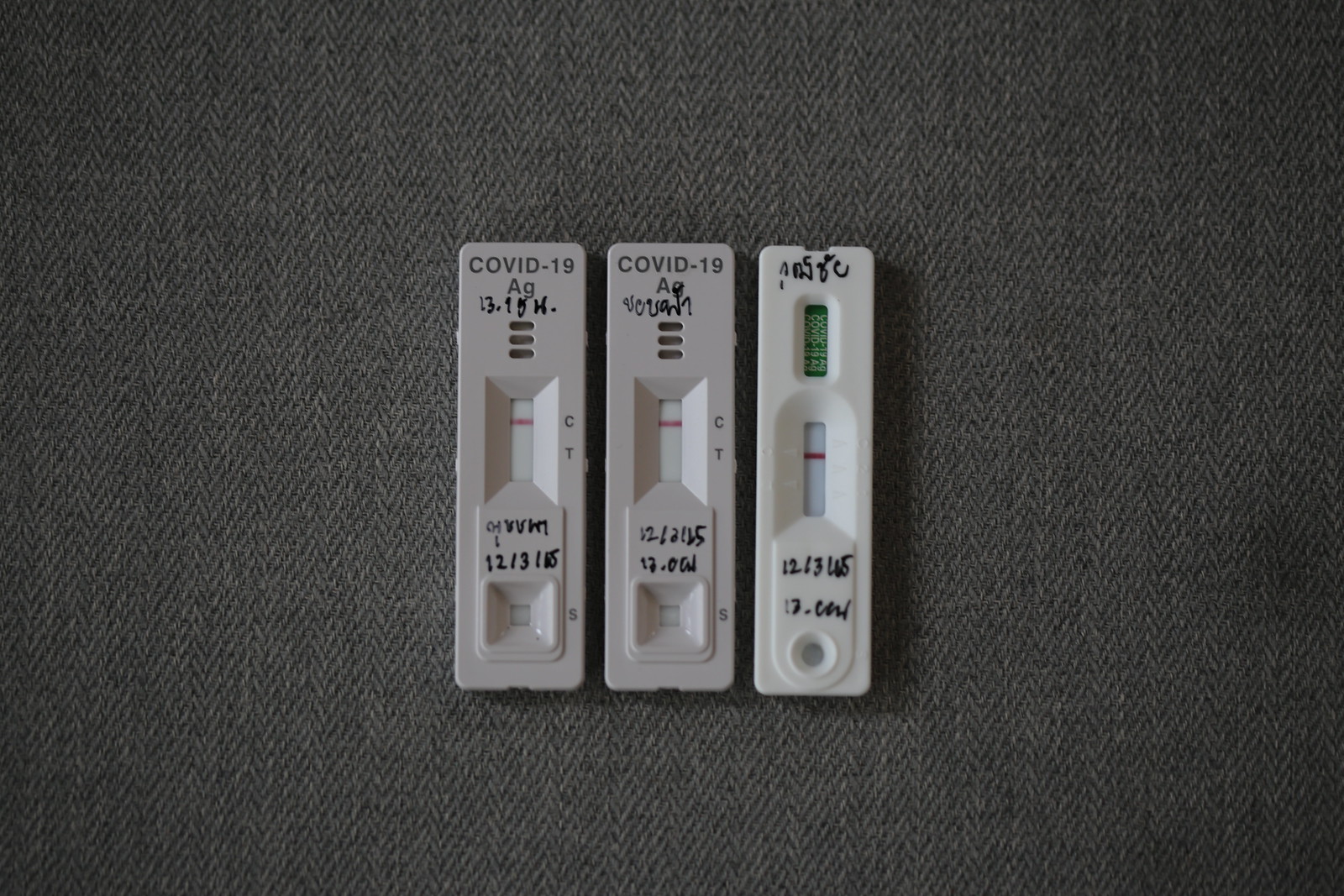The image shows three distinct COVID-19 test kits laid out on a grey surface. Two of these tests appear positive, marked by a red line, while the third test seems to be a different type, featuring a red line as well as a green area in the upper section that the other two lack. The overall color scheme of these tests is muted, with shades of beige, off-white, some green, and red to indicate the test results. The tests are labeled with "COVID-19 AG" along with various unreadable letters and numbers. The dates inscribed on the tests are partially legible, with the first test showing "12.316," the second one "12.2025," and the third one containing text that is not clearly readable. Despite their different visual markers, each test remains housed in a simple, white rectangular box, and all writing is in black, contributing to their bland appearance.